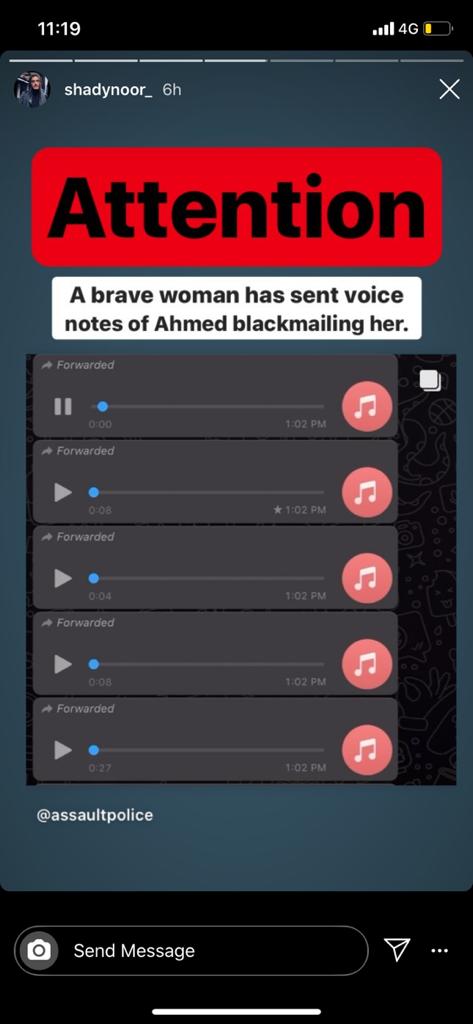Here is the cleaned-up and detailed caption for the image:

---

The image captures a screenshot of an Instagram post sent six hours ago. At the top, the phone displays the time as 11:19 with full bars of 4G connectivity, though the battery is low at about 20%, indicated by a yellow bar. The Instagram interface has a black background, while the post itself is set against a darker blue background.

The post includes a rectangular message with the heading: "Attention: A brave woman has sent voice notes of Ahmed blackmailing her." Below this warning, there are five forwarded voice messages, with the first one currently playing. All these voice messages were sent at precisely 1:02 PM.

At the bottom of the image, there is an '@assaultpolice' tag and a camera icon next to the message input bar. The send button is shaped like a folded paper plane, and a three-dot menu icon is located to its left.